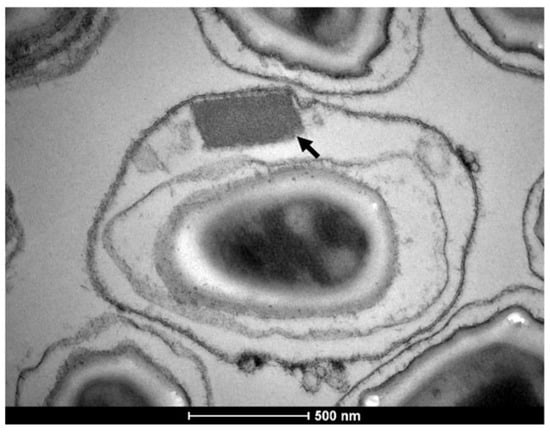The image appears to be taken from a microscope, showcasing what seems to be a cell or a similar microscopic structure on a medium gray background. The focal point is a prominent, oval-shaped form reminiscent of an avocado lying on its side, with a wavy, uneven border. Surrounding this main structure are parts of several other similar cells, all partially visible. At the center of the image is the main oval-shaped cell, containing a dark black-and-gray central area, akin to an avocado pit, encircled by a lighter gray ring, resembling the flesh of the fruit.

The outermost border of the cell is darker, suggesting a membrane-like structure, with a clear, uneven peripheral border. An arrow points to a rectangular gray box located at the top within the largest outer circle of the cell. Below the image, a thin black horizontal bar is present, labeled with "500 NM" and flanked by small, perpendicular white lines, serving as a scale marker. This highly detailed and meticulously captured microscopic view provides a vivid representation of the intricate details of the cell or structure being observed.